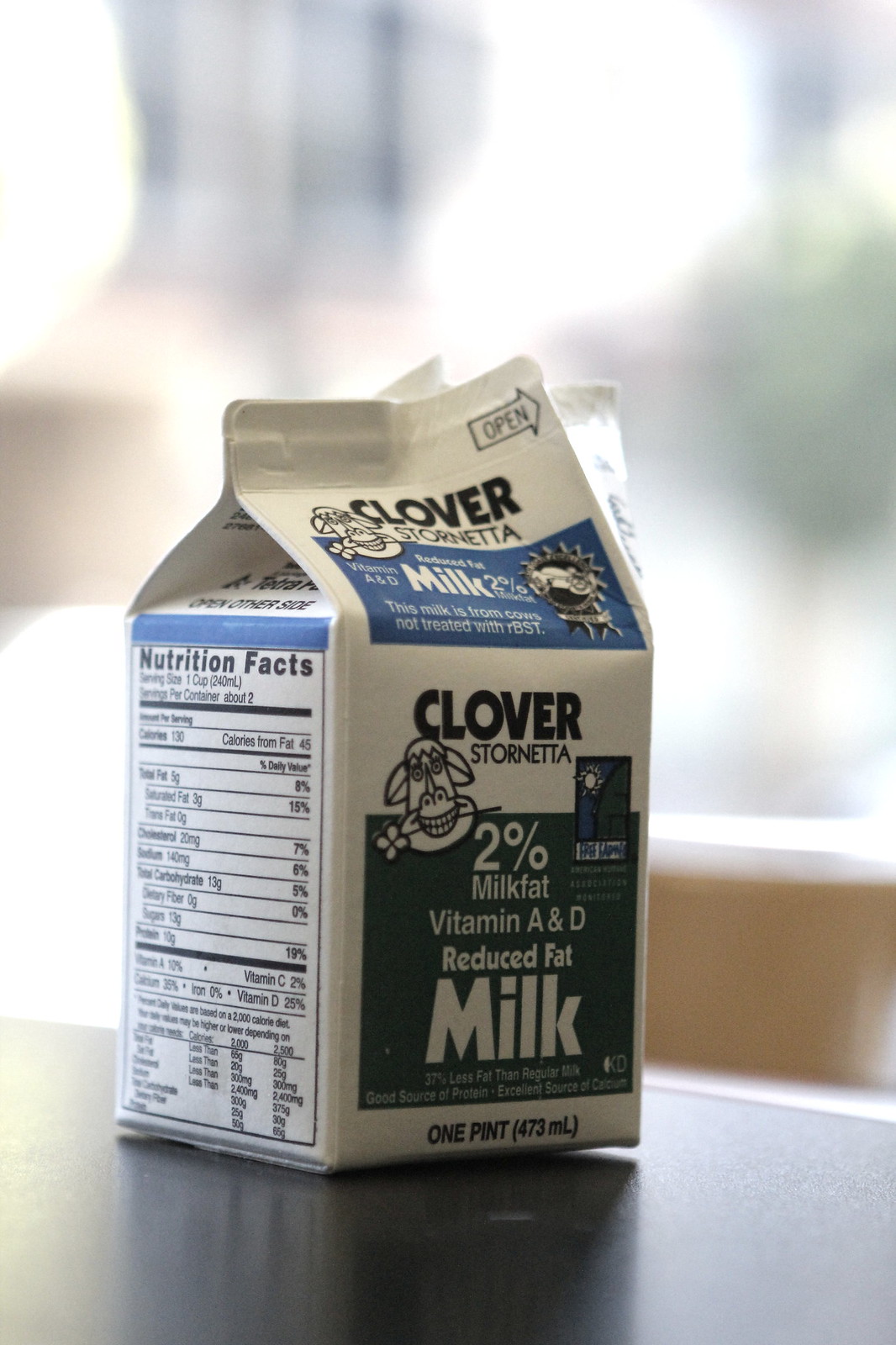The image is a detailed photograph of a small milk carton, resembling those commonly available in school meals. The prominently white and blue carton, branded as Clover Stornetta, features a whimsical illustration of a cartoon cow holding a flower in its teeth, drawn with such detail that its open mouth and hanging ears are visible. This carton prominently displays information about its contents: 2% milk fat, vitamins A and D, and indicates it is reduced fat milk. The carton is positioned on a black or gray surface, with a severely blurry background that may vaguely suggest a building and a tree. The carton is open, showcasing an open notification with an arrow at the top, and the spout faces slightly away from the camera, turned slightly to the back and right. Additional details include nutritional facts on the left side and at the very bottom the measurements, one pint (473 milliliters). An additional face of a character with black spikes on its head is also visible on the top arch of the carton.